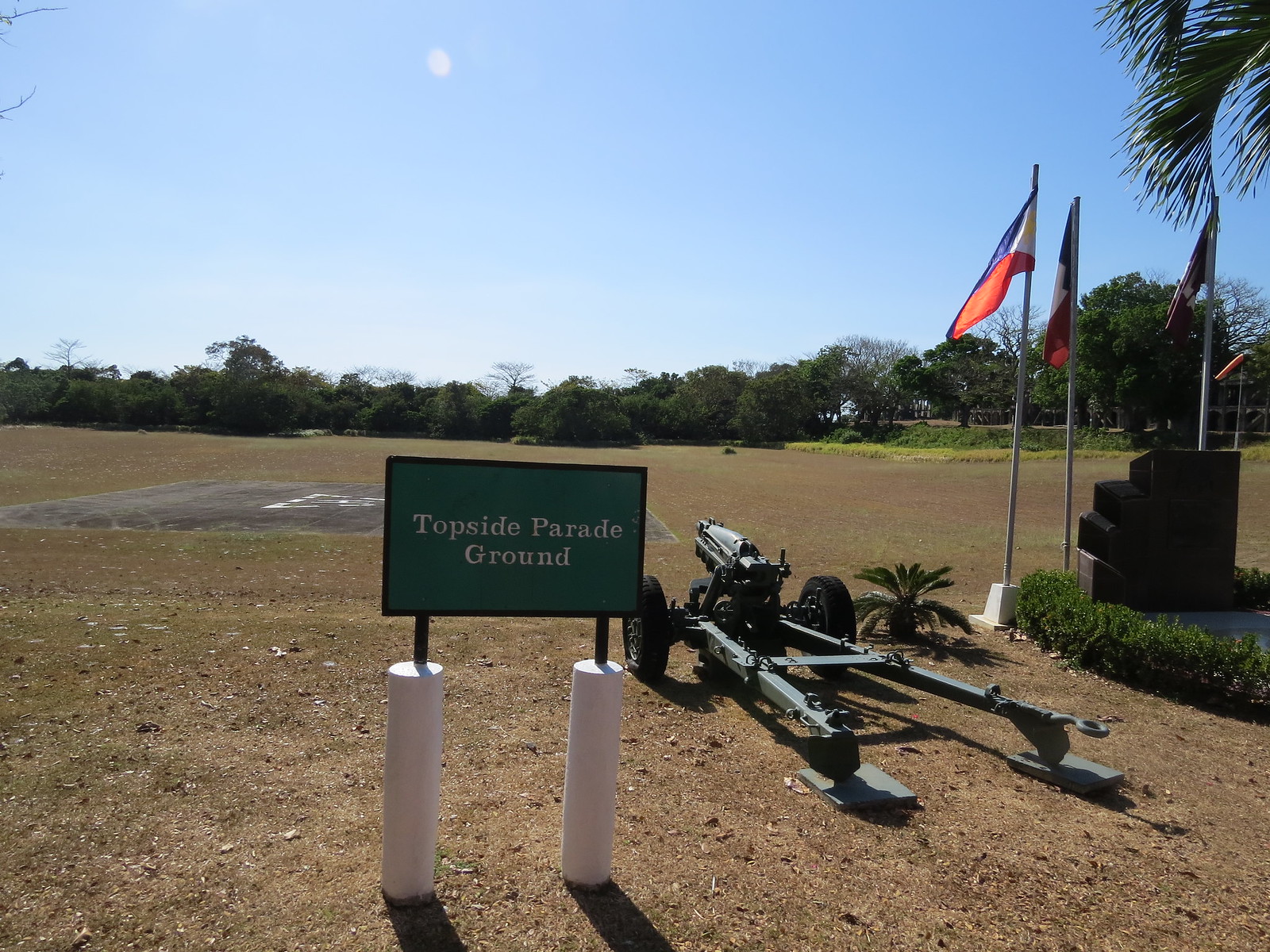The image depicts a vast military parade ground under a clear, light blue daytime sky that fades to white near the horizon. In the distance, a dense line of trees with lush green leaves serves as a backdrop. Closer to the viewer, the ground is covered with a mix of brown and green, neatly cut grass. Prominently in the foreground stands a modern, green-painted military cannon with two large black wheels, pointing toward the tree line. Beside the cannon are flagpoles with blue, white, and red flags, accompanied by small shrubs and plants. A square cement platform with white numbers painted on it is also visible. At the very front of the image, a sign supported by two cement poles reads "Topside Parade Ground."